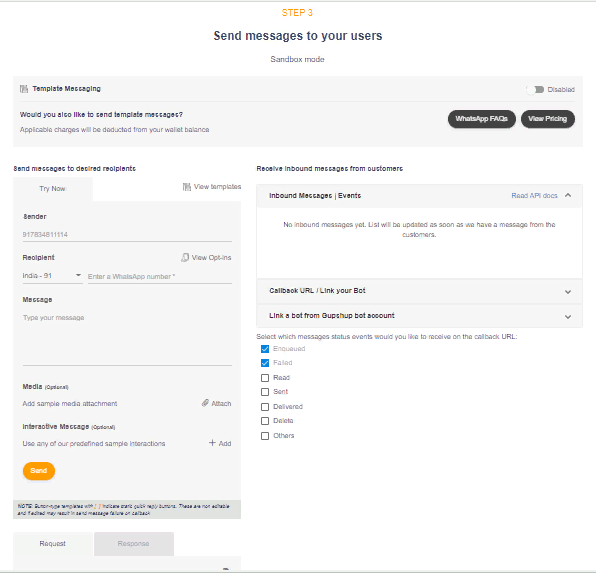The image features a user interface for sending messages, with various instructions and toggles. At the top, there is a grey strip displaying "Template Messaging" on the left side, accompanied by a toggle switch on the right side that is switched off, labeled "Disabled." 

Below this, a title in orange reads "Step 3." Underneath is a black-text instruction stating, "Send messages to your users." Further down, there's text indicating "Sandbox mode."

A grey separator line divides these sections, and below it, there is a prompt asking, "Would you also like to send template messages?" Clarifying this, a note informs users that "Applicable charges will be deducted from your wallet balance." To the right of this message, there are two clickable options: "WhatsApp FAQs" and "View Pricing."

Towards the bottom left, two black buttons with white text are visible. One button instructs, "Send messages to desired recipients," and the other button encourages users to "Try Now." Below these buttons, there is an option to select or enter a sender number, currently showing "Sender: +91 917834811114." 

Additionally, there is a pull-down menu to select the recipient's country (defaulting to "India +91") and fields for entering the recipient's WhatsApp number and typing the desired message.